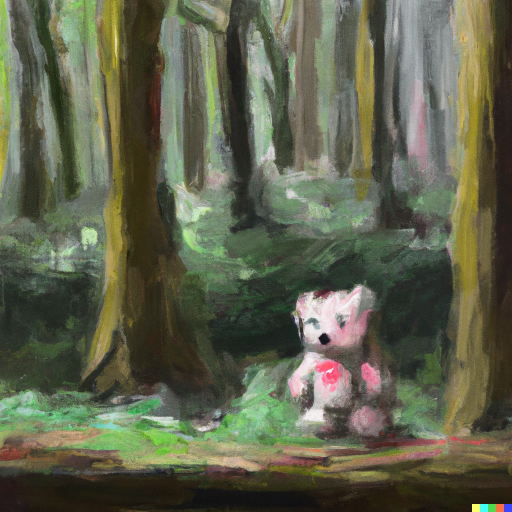The image depicts an impressionist-style painting of a forest scene that is slightly taller than it is wide. Dominated by tree trunks that stretch upward beyond the frame, the foreground features dark and light brown tones with suggestions of flowing grass and brush. A prominent feature is a white teddy bear with pink and red smears, sitting on what appears to be a road or path in the front of the painting. The bottom right corner of the image displays the DALL·E logo, represented by five tiny squares in the colors yellow, cyan, green, red, and navy blue, confirming the image was generated by AI.